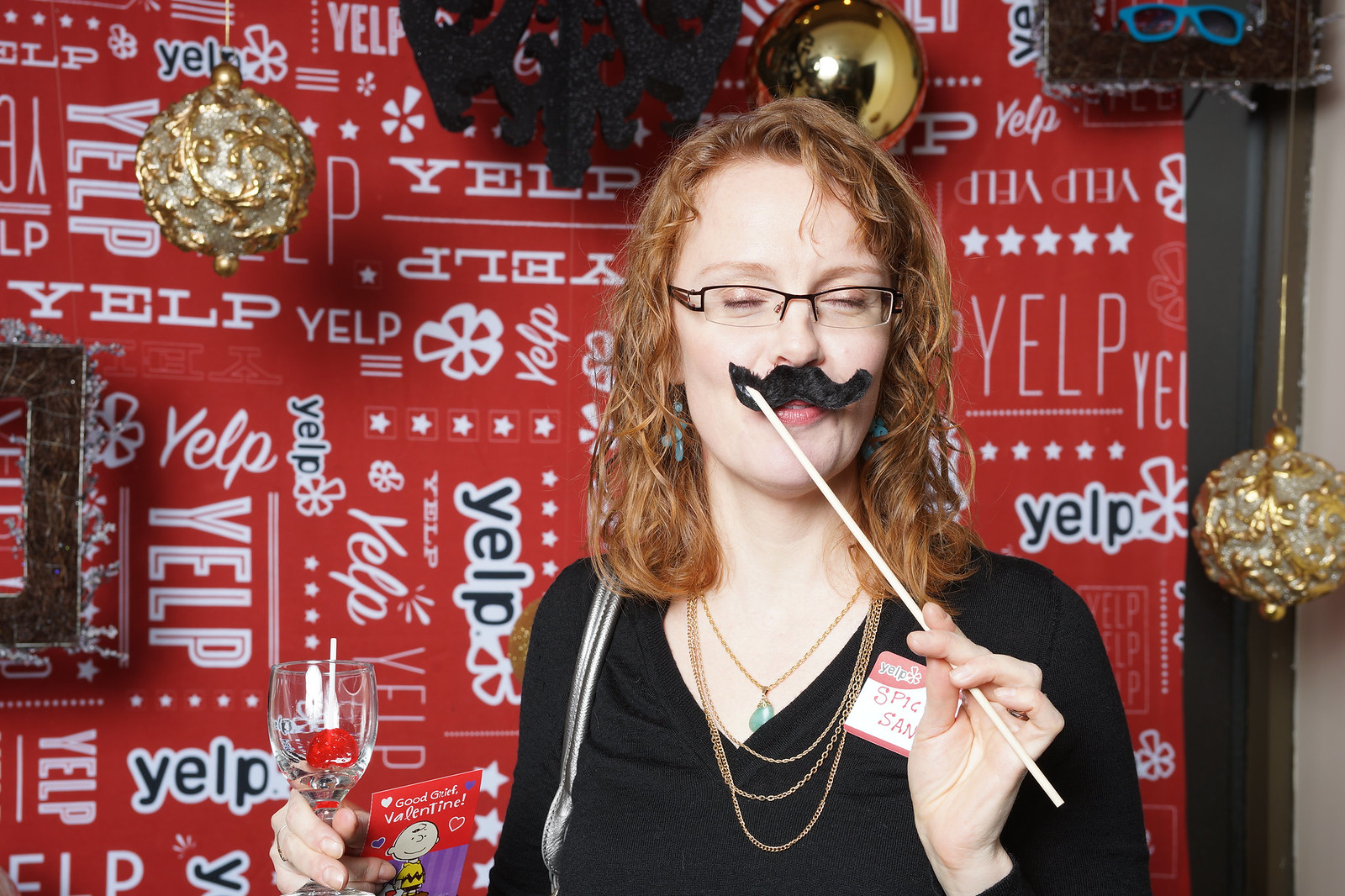In the image, a woman with shoulder-length red hair is depicted at a Yelp Christmas party, standing against a backdrop adorned with repeating Yelp logos. She sports a fake mustache in a Charlie Chaplin style, held in place with a stick while her eyes are closed and she wears glasses. Dressed in a black v-neck outfit, she accessorizes with multiple strands of gold necklaces and a stone pendant. A name tag on her attire reads "Spicy Sam." Additionally, she's seen holding a glass of white wine in one hand, while a Charlie Brown Valentine’s card is also part of the scene. The festive atmosphere is enhanced by visible Christmas decorations, contributing to the indoor event's celebratory ambiance.